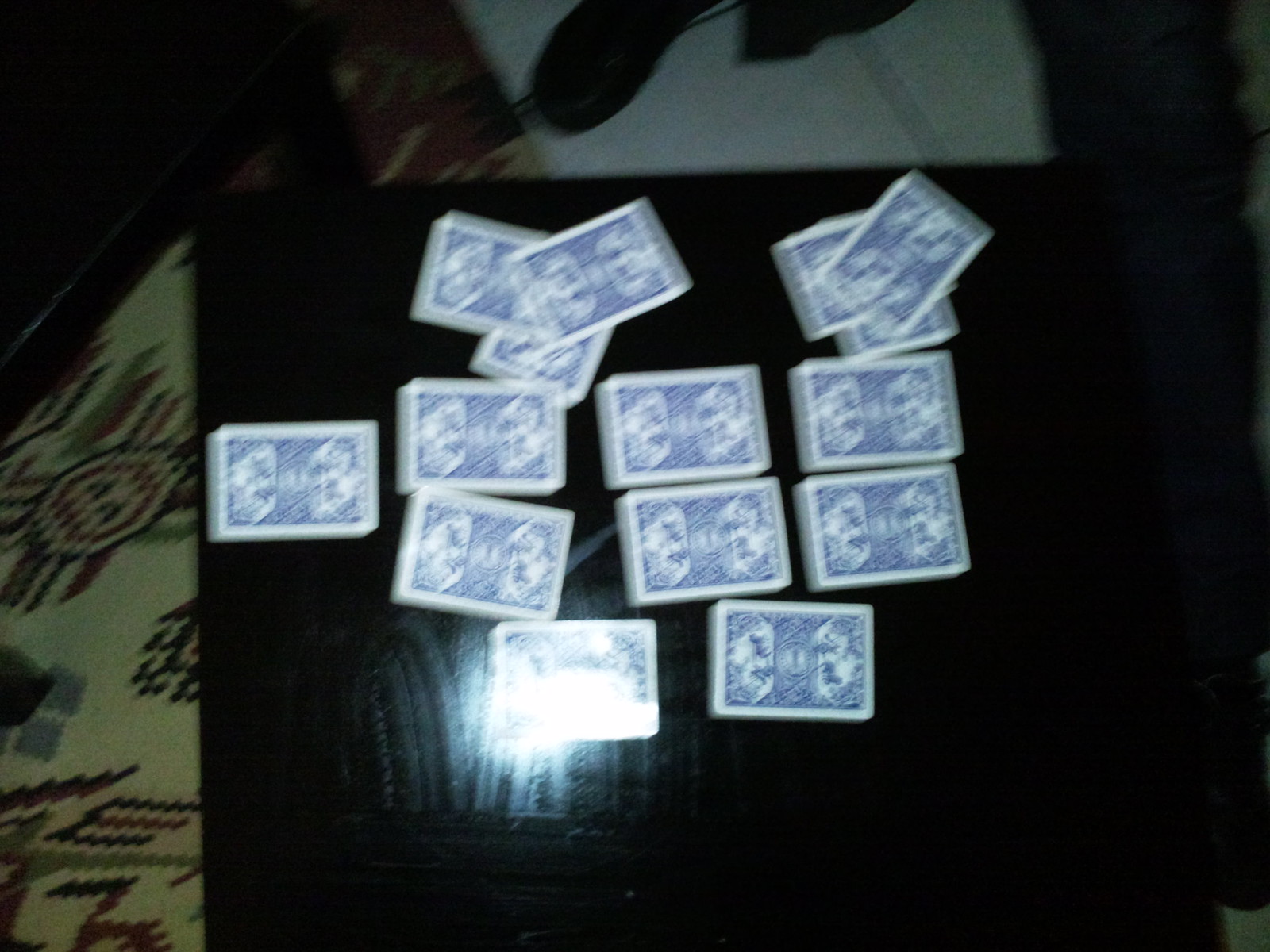This indoor color photograph offers a bird's-eye view of a black wooden coffee table positioned diagonally across the lower two-thirds of the frame. The table’s surface is scattered with approximately 13 to 14 playing cards, all face down and adorned with a blue design. Due to the blurred quality of the image, the finer details of the cards remain unreadable. Most cards are oriented horizontally, with a few lying diagonally, suggesting a casual, unstructured arrangement rather than an ongoing game. 

In the background, occupying the upper third of the image, is an area rug showcasing a vibrant Aztec pattern. The rug's design features white, tan, red, green, and brown hues in traditional geometric motifs. In the upper right corner, part of a tiled floor is visible, contrasting the elaborate rug pattern.

A noticeable flash glare is present slightly left of center in the lower half of the photo, reflecting off the black table surface. There also appears to be a faint, black outline of what might be a person's foot encroaching from the middle top edge of the image, adding an ambiguous human element to the scene.

The overall ambiance is one of casual disarray, reflected in the random scattering of cards and the lack of any discernible text or printed material within the photograph.